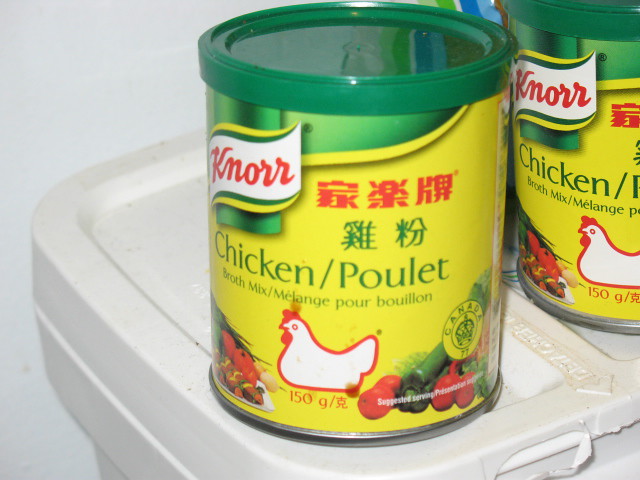The image showcases two jars of Knorr chicken bouillon, arranged on a white plastic surface. Each green jar features a prominent yellow label. The front jar is fully visible, while only half of the front of the adjacent jar is seen. The yellow label is dominated by the Knorr logo, characterized by a red cursive script set against a white background with green and yellow accents. Below the logo, the label contains red and green text in Japanese or Chinese, as well as the English and French wording "chicken/poulet, broth mix, mélange pour bouillon." An illustration of a chicken and various vegetables adorns the bottom of the label. The jars are topped with green lids, resembling those of coffee containers, and each jar contains 250 grams of the product.